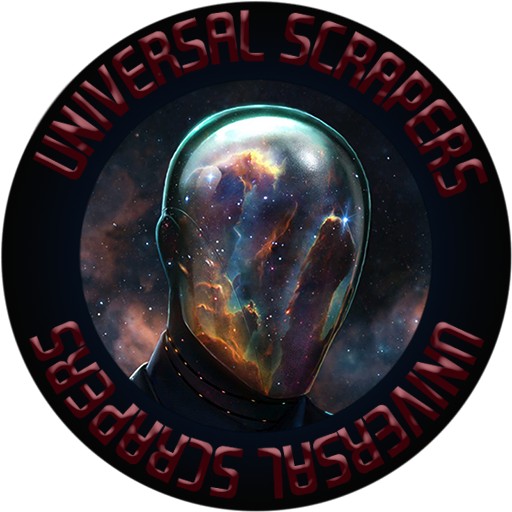The image depicts a logo for "Universal Scrappers," encapsulated within a black circular background. Prominently placed at the top and bottom of the circle is the brand name "Universal Scrappers," written in a deep maroon, shiny text that appears slightly raised. The text at the bottom is upside down, mirroring the top. Inside the circle, there is a stylized depiction of a head and shoulders, though the face is replaced by a reflective globe, mirroring an expansive view of space, including a nebula and celestial bodies. The neck and shoulders are rendered in black, blending seamlessly with the background, and only one ear is visible. The overall design suggests a futuristic or space-themed company logo, with a striking emphasis on the cosmic imagery reflected in the face, reminiscent of a space helmet.